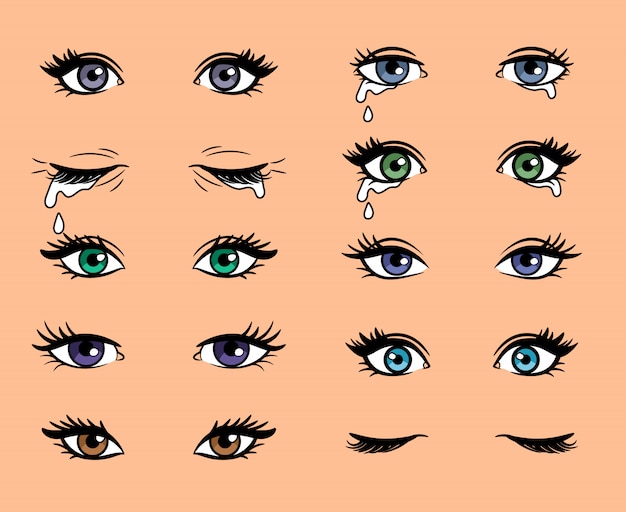This illustrated image showcases a diverse array of animated human eyes against a skin-tone colored background. There are ten pairs in total, each varying in color, size, and expression. The eye colors include two rich green, two striking purple, one vivid turquoise blue, two neutral gray, and one warm brown. Two sets of eyes are closed; one appears to be shut tightly, while the other looks like it's crying. Among the open eyes, expressions range from emotional and teary to flirty and bored. The eyes also differ in shape and detail, especially in the styles of their eyelashes, adding to the overall variety and richness of the depiction.